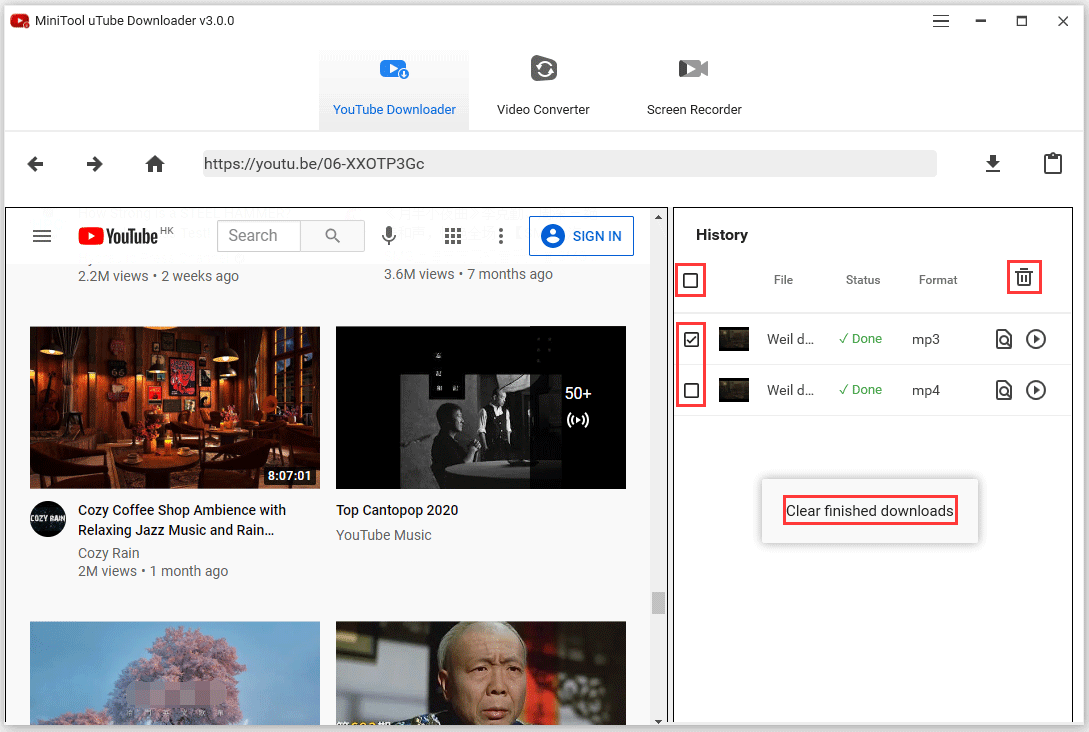Caption: "This detailed screenshot appears to be taken from a YouTube page interface within MiniTool YouTube Downloader v3.0.0. At the top left corner, the application name is displayed. Three main functions are available for clicking just below: 'YouTube Downloader,' highlighted in blue, 'Video Converter,' and 'Screen Recorder.' A search bar in the main window has a pre-typed YouTube channel. Underneath the search bar, there's another YouTube icon and a list showcasing four different video options from the channel. The visible titles are 'Cozy Coffee Shop Ambience with Relaxing Jazz Music and Rain' and 'Top Cantopop 2020 YouTube Music,' each accompanied by a thumbnail image. The bottom two video thumbnails are partially cut off, one showing a mix of blue and pink colors, and the other featuring an older man with short hair. To the right, there's a history section labeled 'File,' 'Status,' 'Format,' and a trash icon. Two workflows are marked as 'Done,' one corresponding to MP3 and the other to MP4 formats. An option labeled 'Clear Finished Downloads' is available at the bottom of this panel."